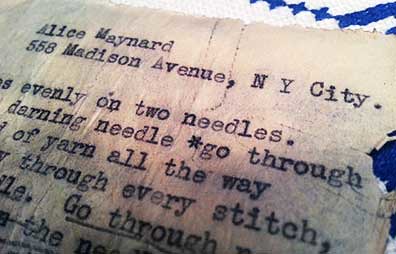This image shows a slightly angled, weathered, and vintage piece of paper, possibly dating back a few decades. The document appears to have been typed using an old-style typewriter with black ink, presenting the recipient's address prominently at the top: "Alice Maynard, 558 Madison Avenue, New York City." The text below includes incomplete instructions related to darning needles and yarn, indicating it might be a manual or note, perhaps for a factory worker. The white but age-worn and off-white paper is damaged, with noticeable tears along the right edge. In the background, there is a fabric with a blue and white star-like pattern in the top right corner, adding a subtle yet distinct color contrast to the otherwise monochromatic document. The photograph captures the document in a realistic, representational style, emphasizing the tactile and historical essence of the paper.